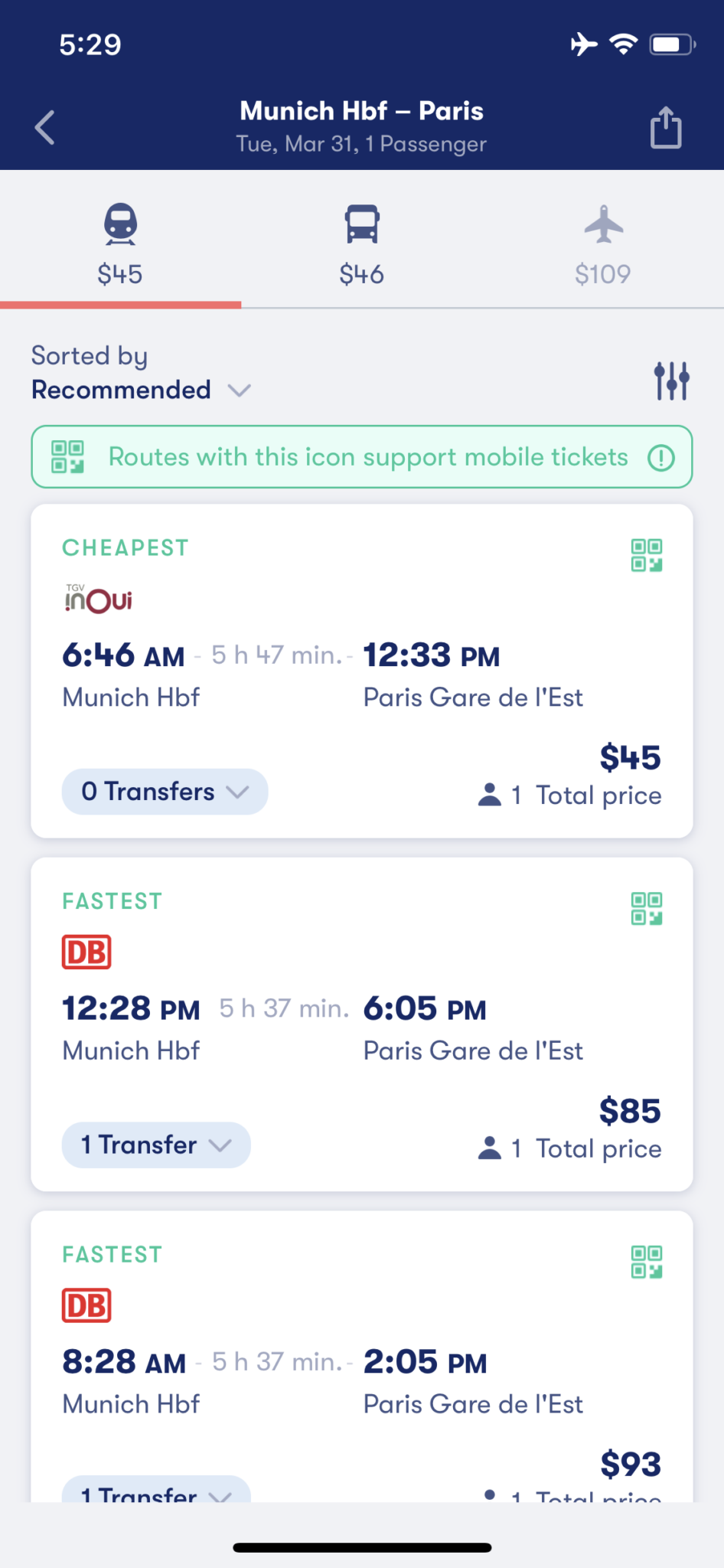**Detailed Caption:**

This image is a screenshot from a mobile phone displaying detailed travel information for a trip from Munich HBF to Paris. The interface features a dark blue header, which prominently displays the travel route "Munich HBF - Paris" at the bottom center. Just below the header, the date "Tuesday, March 31st" and the notation "one passenger" are provided.

Beneath this, three travel options are arranged horizontally with corresponding icons:
1. The first option is high-speed rail, indicated by a train icon on tracks, listed at a cost of $45. This option is currently selected, as denoted by the orange underline.
2. The middle option is a bus, represented by a bus icon, priced at $46.
3. The rightmost option is an airplane, shown by a grayed-out airplane icon, with a fare of $109.

Following the travel options, there is a sorting section labeled "sorted by recommended," accompanied by a drop-down box on the right side.

Below this section, a prominent green banner informs users that routes with a QR code icon support mobile tickets. 

Under the green banner, three ticket options are displayed within white boxes:

1. **First Ticket Option:**
   - Top-left corner labeled "cheapest" in green.
   - A QR code to the right.
   - Details include train name, departure and arrival times, with a total travel duration of 5 hours and 47 minutes centrally displayed.
   - A drop-down box on the bottom left states "zero transfers."
   - Price listed as $45, with "one passenger" and "total price" below the fare.

2. **Second Ticket Option:**
   - Top-left corner labeled "fastest."
   - Additional details and layout similar to the first option with different specifics for the fastest route.

3. **Third Ticket Option:**
   - Similarly labeled "fastest" in the top-left corner.
   - Follows the same layout structure, presenting specifics for another fastest travel route.

Overall, the screenshot provides comprehensive travel information, enabling users to easily compare different transportation options, fares, and travel durations for a journey from Munich HBF to Paris.